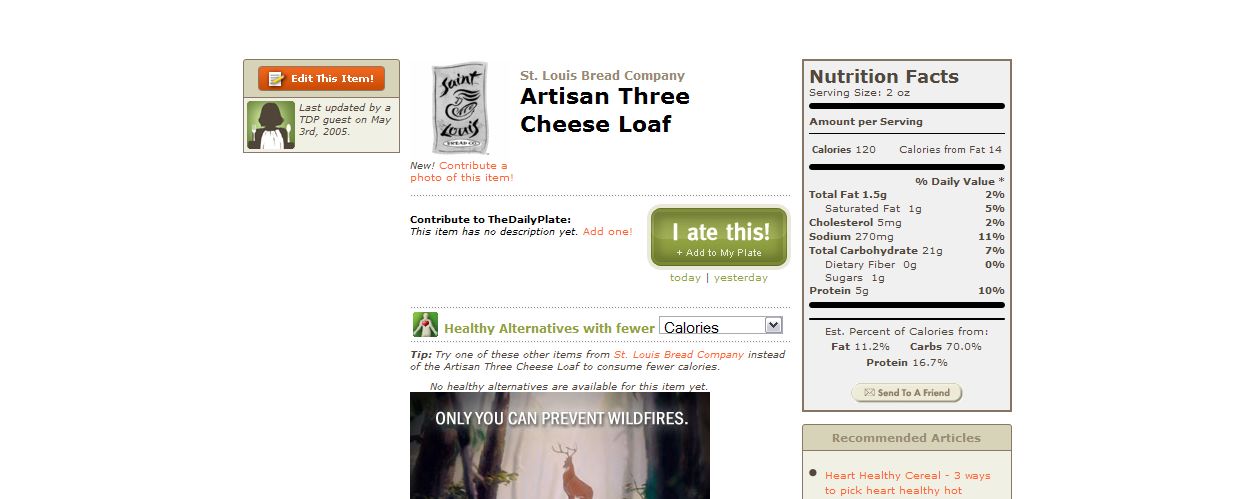In this detailed image set against a stark white background, several elements are presented in a structured format. Starting from the upper left corner, a computer screen displays an icon resembling a personal account, accompanied by text that notes, "Last updated by a guest on May 3, 2005." Adjacent to this, a section reads "St. Louis Bread Company Artisan 3 Cheese Loaf" and prompts users to "Contribute a Photo of this Item." Below, it encourages contributions to the "Daily Plate," indicating that the specific item currently lacks a description but includes the personal note, "I ate this."

Positioned to the right of these elements, a detailed Nutrition Facts label is prominently displayed. It specifies nutritional information for a 2-ounce serving size, noting it contains 120 calories with 14 calories from fat. The label further breaks down the nutritional content: 1.5 grams of total fat, 5 grams of protein, 270 milligrams of sodium, and 21 grams of total carbohydrates. This comprehensive layout appears to represent a calorie and nutritional tracking application, likely aimed at helping users monitor their dietary intake.